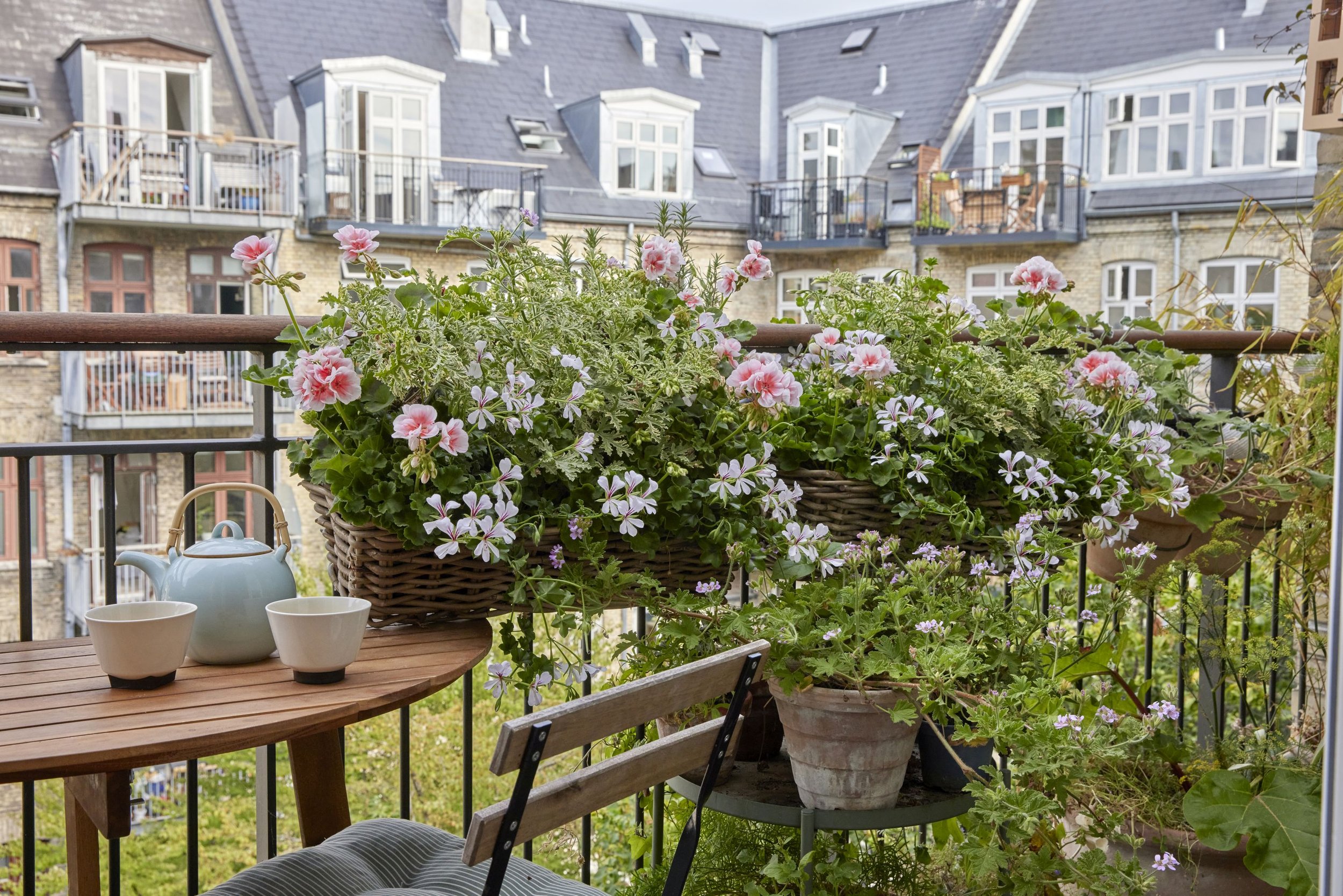This photograph captures a tranquil scene from a European-style apartment balcony. The cozy space is adorned with an array of flowering plants in various planters hanging along the wrought iron railing and a profusion of pink blooms in baskets. Central to the balcony is a wooden bistro table, reminiscent of a design seen at Ikea, featuring a teapot with a gold handle and two matching white teacups, inviting a moment of relaxation. A comfortable brown chair with a white cushion complements the setup. In the background, the view extends to neighboring apartment buildings made of brownish-yellow brick, some with white framed windows while others with brown. The steep, slate gray roofs and multiple balconies add to the Parisian ambiance. Below, a lush grassy courtyard connects these buildings, enhancing the European feel of the entire scene.